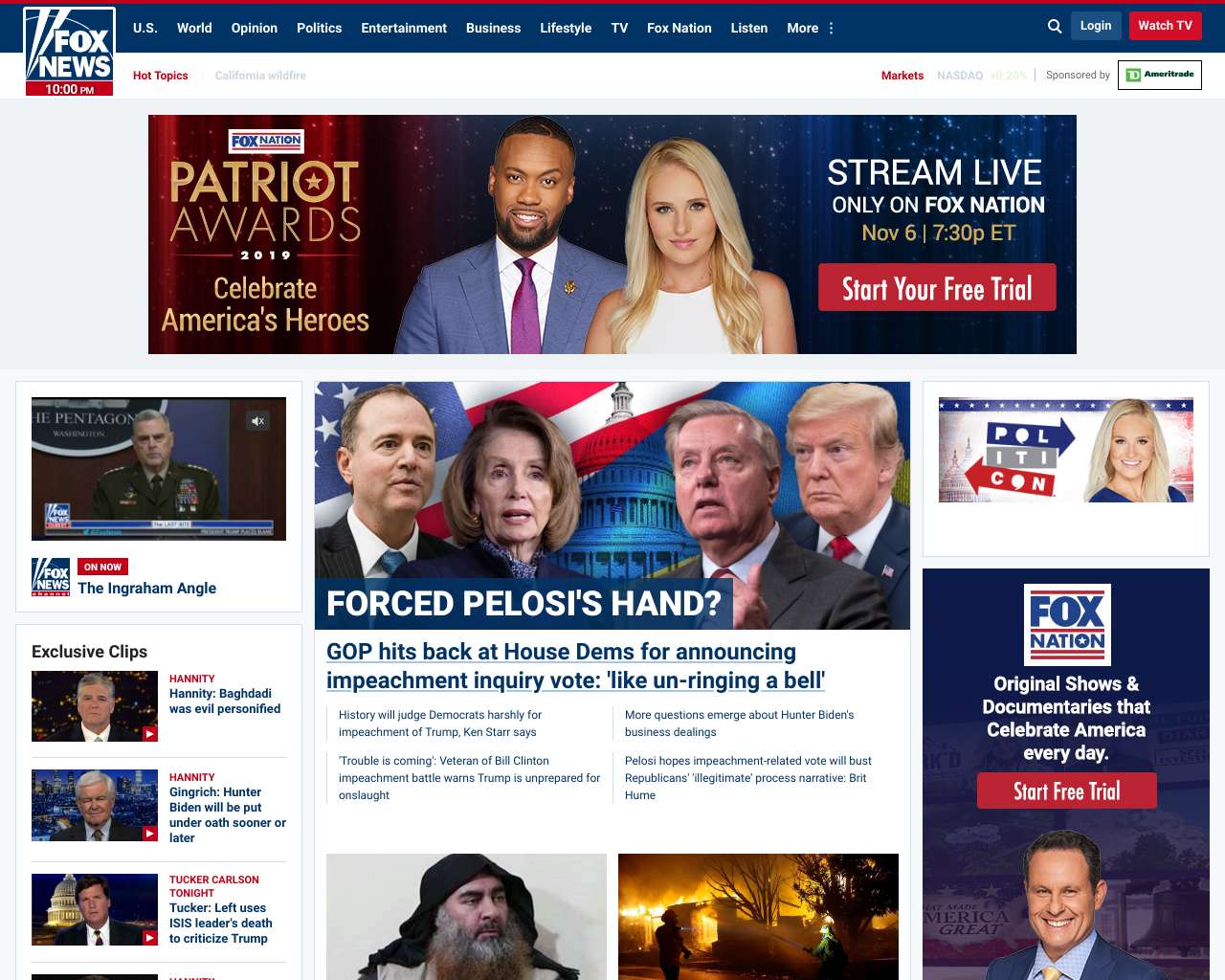This screenshot captures the homepage of Fox News at precisely 10 PM. The top section prominently features the Fox News logo with a row of navigation tabs beneath it, including categories like US, World, Opinion, Politics, Entertainment, Business, Lifestyle, TV, Fox Nation, Listen, and More, with an additional three-dot menu for extended options. A search icon, login button, and "Watch TV" button are also visible.

Directly below the main navigation is a "Hot Topics" bar highlighted in red. Adjacent topics include "California Wildfire" in white and "Markets" in red, followed by "NASDAQ," displaying a positive increment of +0.20%, and a note stating "Sponsored by TD Ameritrade."

The middle section showcases a large banner promoting the Patriot Awards 2019, encouraging viewers to "Celebrate America's Heroes" with two anchoring figures pictured. It details streaming live only on Fox Nation, set for November 6 at 7:30 PM Eastern, alongside a call-to-action to "Start Your Free Trial."

Further down, several different news stories and exclusive clips are displayed. A bold banner with the headline "Force Pelosi’s Hand?" captures additional viewer interest. Adjacent tabs about current events, such as the California Wildfire and Politicon, along with various advertisements, complete this dynamic homepage snapshot, which focuses heavily on content available through Fox Nation.